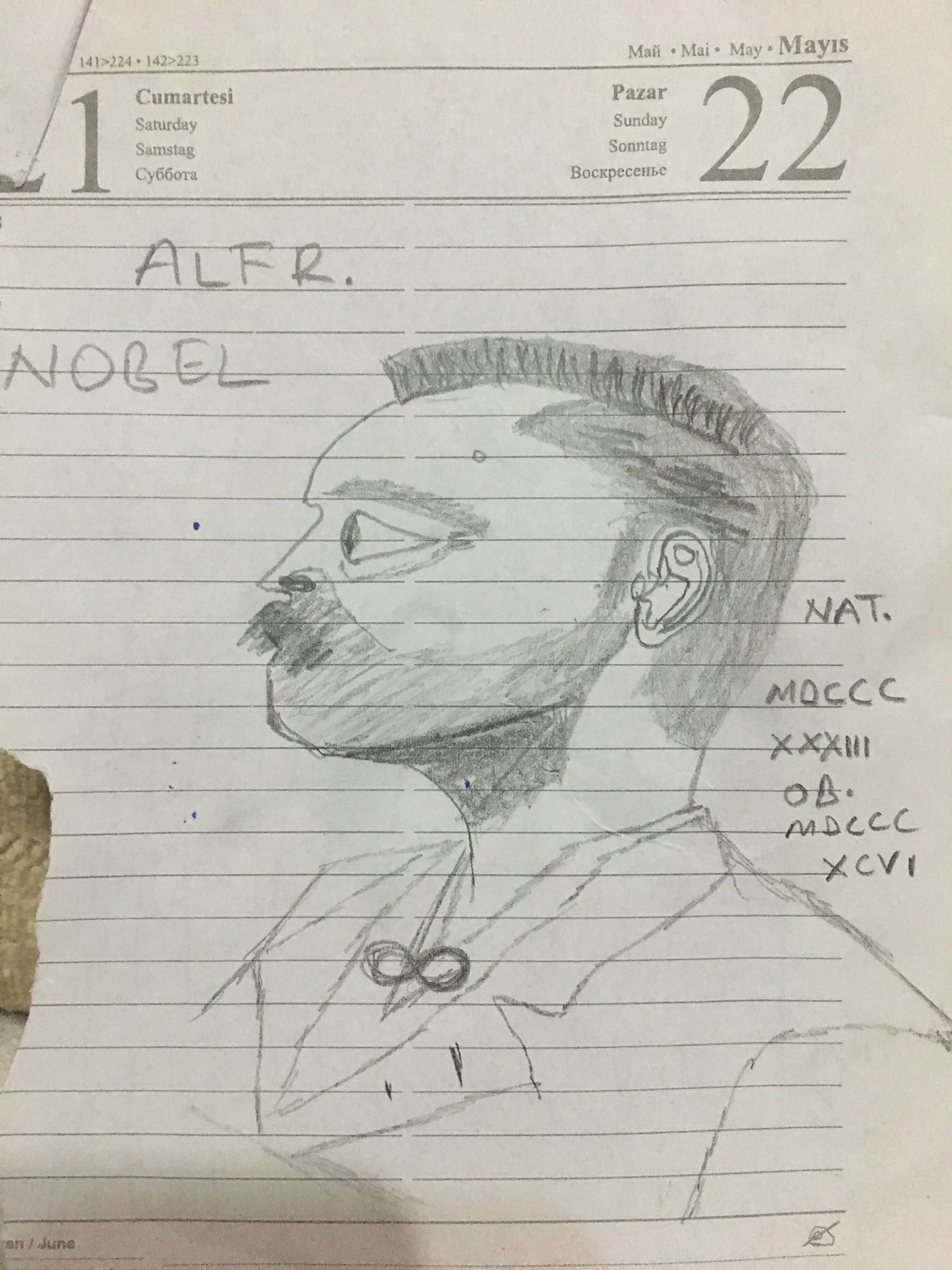This image showcases a detailed pencil drawing on a lined piece of school notebook paper, portraying the left-side profile of a man. The man has short, spiky hair at the top, a thick mustache, and a close-cropped beard. He is dressed in an old-fashioned suit with a bow tie. The portrait is refined with a pointed nose and a dignified appearance, though it is primarily drawn in outline form. At the top left corner of the paper, which seems to resemble a daily planner or calendar page, there is printed text in colored ink indicating the days "Saturday" and "Sunday" with the numbers "21" and "22" respectively, hinting at the dates within May. Additional notations in pencil include the name "ALFR dot Nobel" near the top, suggesting that this might be an artistic interpretation of Alfred Nobel. To the right of the man's profile, there are enigmatic Roman numerals: "NAT MDCCCXXXIII" and "OB MDCCCXCVI," potentially indicating birth and death years. Notably, the drawing lacks an artist's signature.